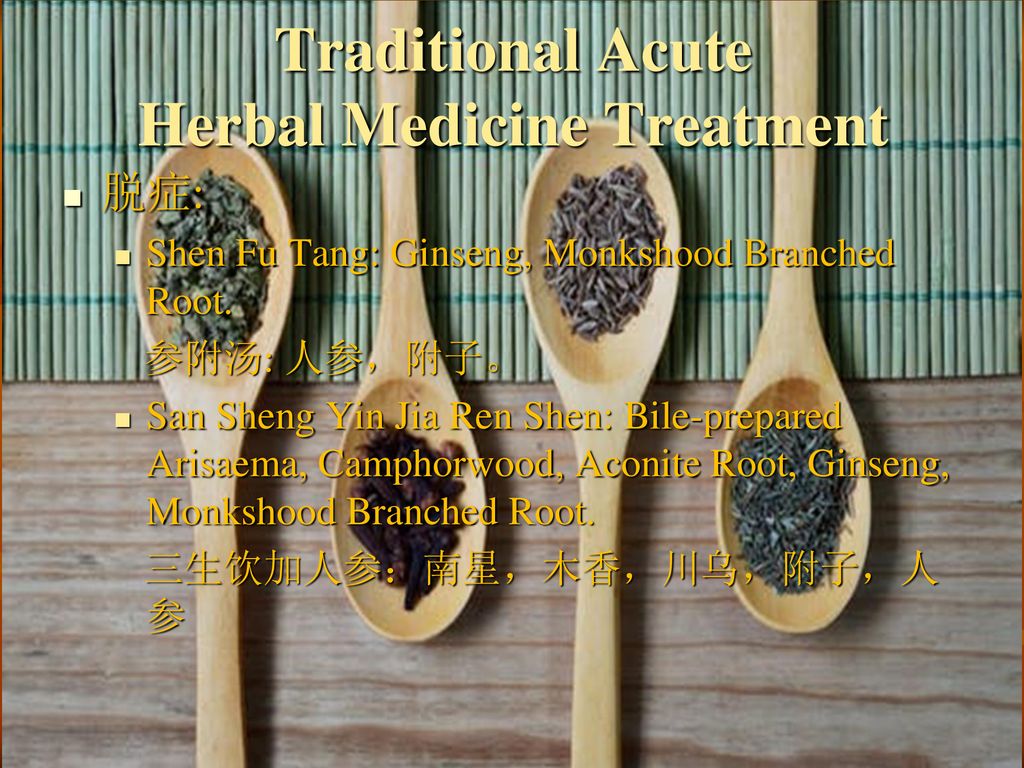This color photograph captures four wooden spoons arranged on a two-tone background, transitioning from a sage green mat at the top to a light wooden tabletop at the bottom. Each spoon, positioned in alternating directions, contains small, granular items representing various Chinese herbs. At the top of the image, the text "Traditional Acute Herbal Medicine Treatment" is prominently displayed in light yellow. Below this, multiple lines of Chinese characters are interspersed with English translations. The translations list specific herbal preparations including "Shen Fu Tang, Ginseng, Monkshood, Branched Root," "San Sheng Yin Jia Ren Shen, Bio-Prepared Arisaema, Camphor Wood, Aconite Root, Ginseng, Monkshood, Branched Root." The detailed arrangement and labeling suggest the image showcases different herbs and their respective uses in traditional Chinese medicine.